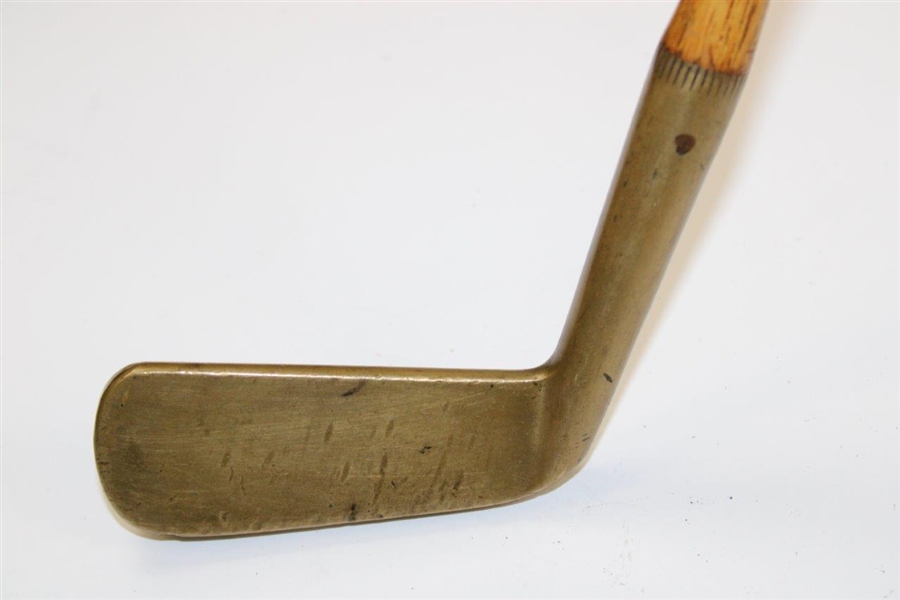The image features an up-close view of an old-fashioned golf driving iron, prominently displaying the head of the club and a small segment of the shaft. The background is an unembellished off-white or very light gray, ensuring full focus on the club itself. The head of the iron, made of dark olive or bronze-colored metal, shows extensive use, evidenced by numerous scratches, scuff marks, and one distinctive black spot near the stick. The metallic surface also has patches of silver and brown from wear and tear. The shaft extends from the head and is made of a light orange-ish brown wood, visible only at the top right edge of the image, suggesting it continues beyond the frame for the golfer to hold.